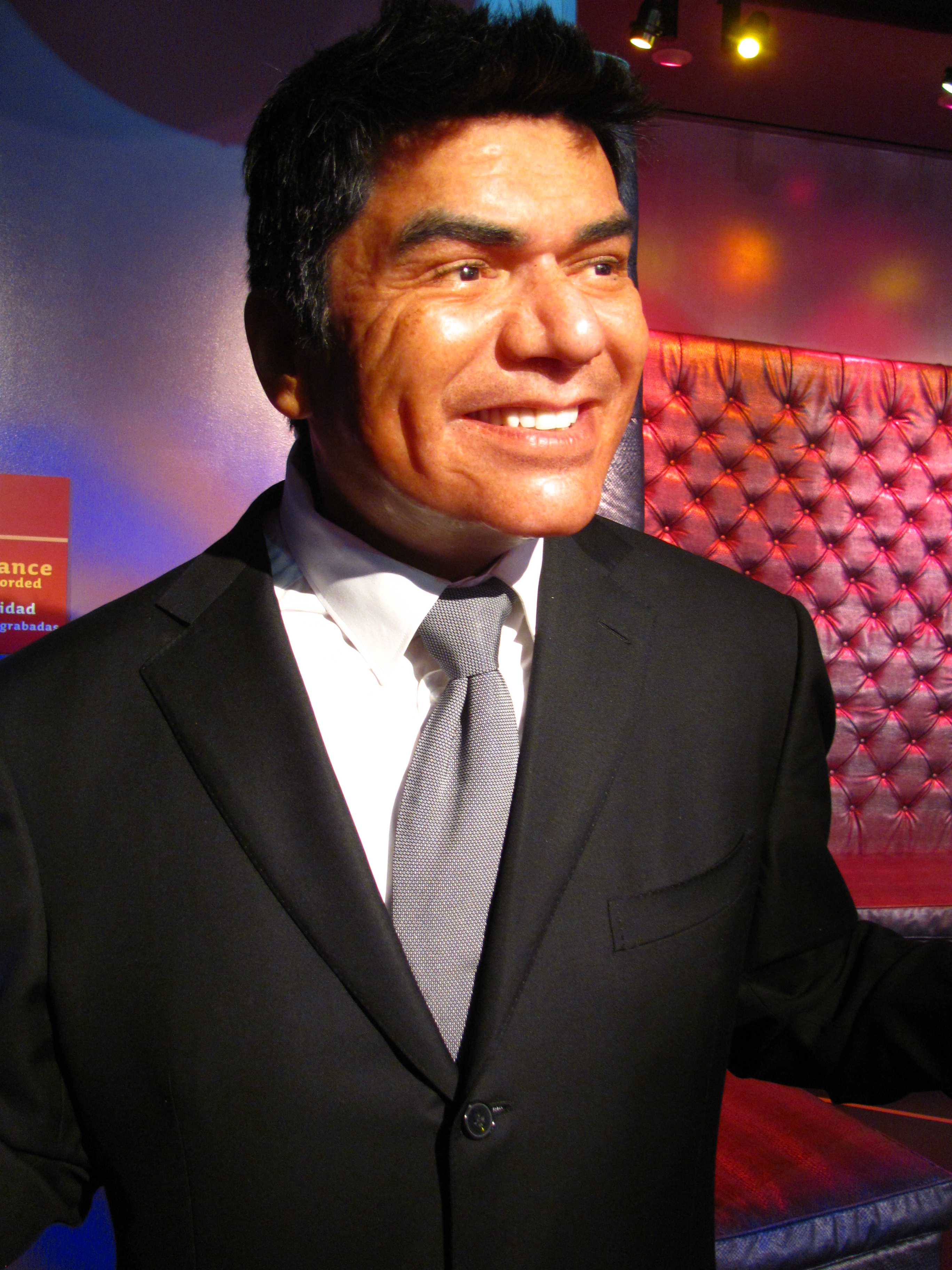The image features what appears to be the wax figure of George Lopez, the famous Hispanic-American comedian and TV personality, known for his classic salt-and-pepper hair and signature smile. Dressed in a modern black suit with a silver tie and a shirt, he stands serenely on a stage resembling a set from a comedy show, complete with a dark redwood floor and a plush, velour-cushioned red wall to the right. The scene is bathed in colorful stage lights that give the photograph a warm, reddish hue. The figure's detailed facial features, including his expressive eyes and the iconic wrinkles that form when he smiles, further suggest a lifelike representation typically found at places like Madame Tussauds. The intricate tie pattern is nearly reminiscent of television static, adding to the lifelike quality and contemporary styling.